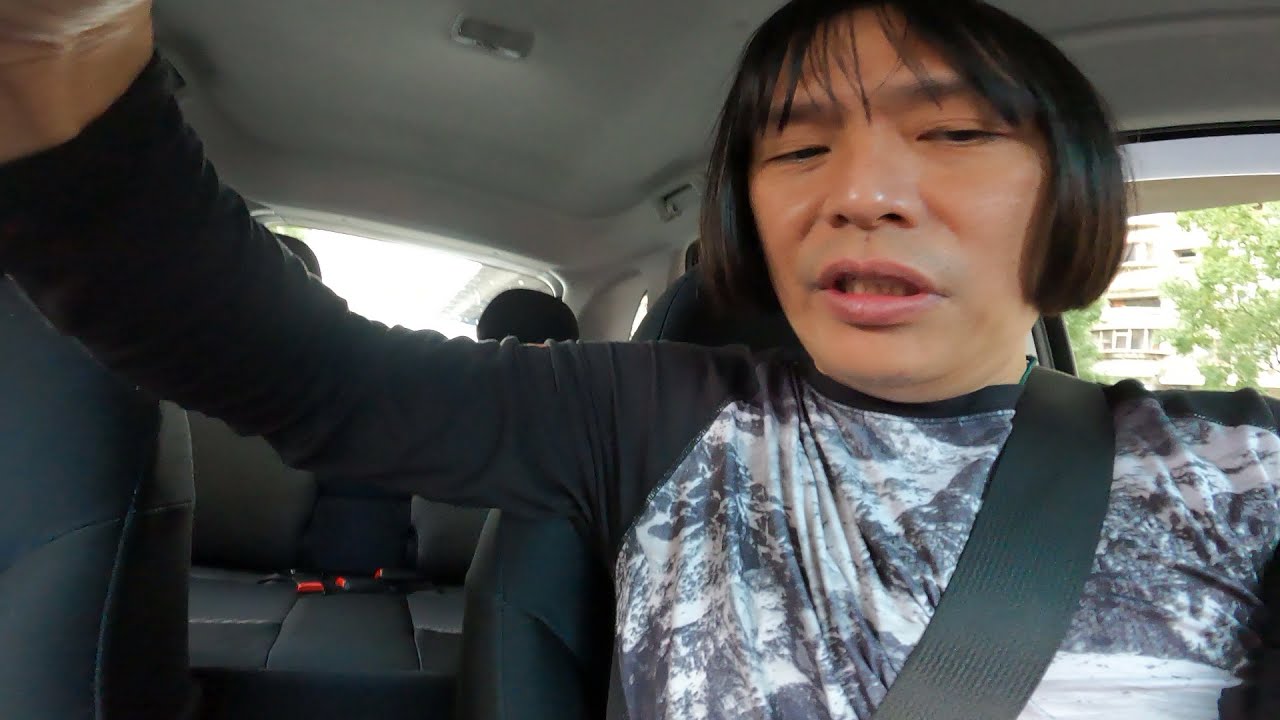The image features a young male with short, dark black hair that has faint highlights, styled in a mushroom or bowl cut. He is sitting in the driver's seat of a car, strapped in with a black seatbelt. He wears a long-sleeved black shirt with gray or white patterned art on it. His right hand is raised, suggesting he might be about to make a driving motion or interact with the car's controls. His face appears to be squinting with his mouth partially open, and he is looking down at the steering wheel area. 

The car’s interior is predominantly black, with a gray ceiling. There are no visible passengers in the back seat, and the passenger seat is not visible in the image. Out the left side window, one can see a well-lit building, indicating that the photo was taken during the daytime. Additionally, multiple trees with green leaves can be seen outside, enhancing the daytime setting of the photograph. The overall focus of the image is on the man and the car's interior, with clear details on his attire and the surroundings outside the vehicle.